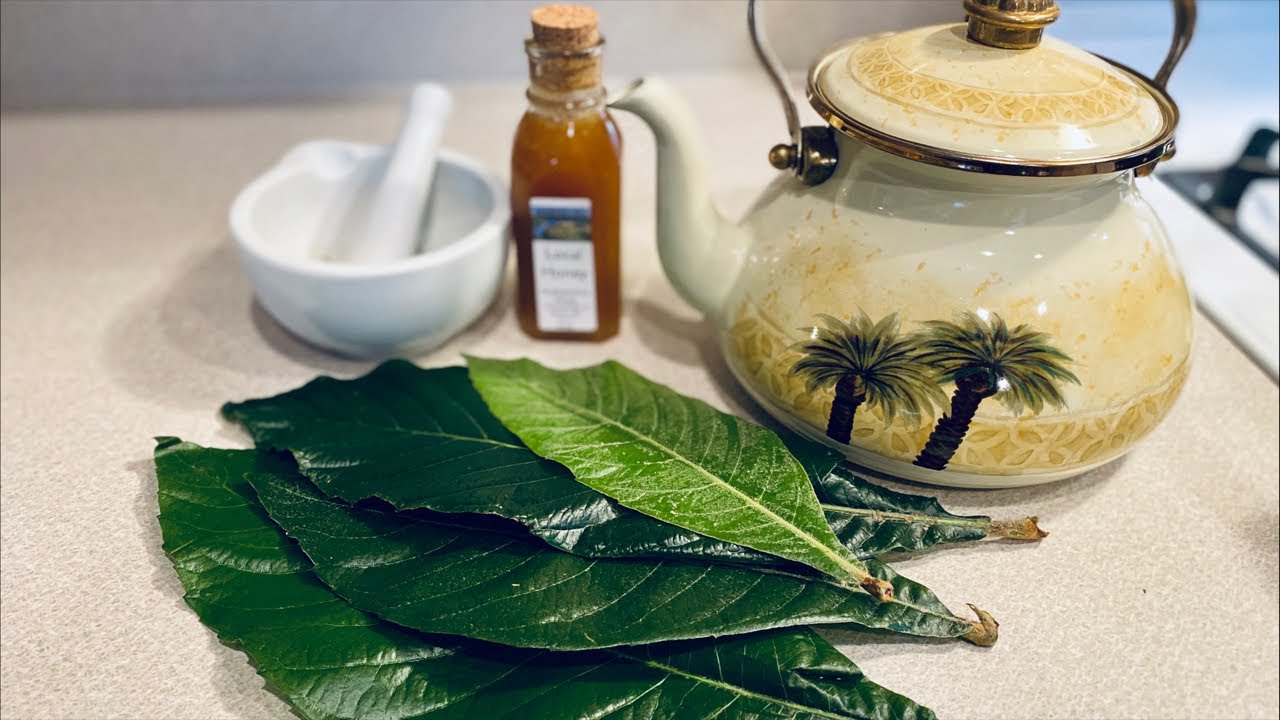In this detailed studio-lit still life photograph, a serene kitchen scene is meticulously arranged on what appears to be a pearly white countertop, adjacent to a blurred gas stovetop. Dominating the foreground, a stack of four large, shiny, mint leaves extends toward the bottom of the frame. Behind this verdant display, slightly out of focus, stands a small, white mortar and pestle, centrally positioned, suggesting its use in grinding fresh ingredients. Immediately to the right, a glass jar filled with a honey-colored liquid, sealed with a wooden cork, adds a warm, inviting tone to the composition. Completing the setup on the upper right side is an off-white teapot adorned with green palm trees and detailed with gold trim, its spout elegantly pointing to the left. The teapot’s subtle dark yellow speckles and golden metal details near the lid enhance the aesthetic charm. This carefully curated arrangement suggests a tranquil moment of preparing a cup of mint tea, sweetened with honey, in an inviting kitchen setting.